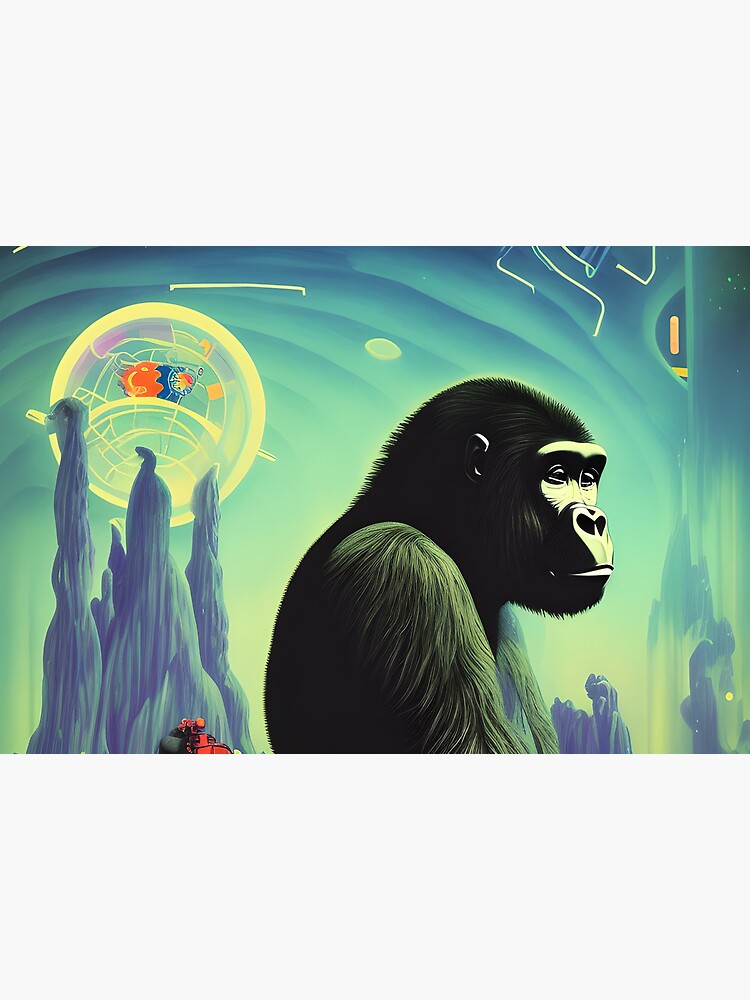This digital art piece, rectangular in shape, depicts a melancholic gorilla-like monkey, akin to King Kong, facing the right. Rendered primarily in black with greenish hues highlighting parts of its upper body, the creature's detailed face shows ears, eyes, nose, and mouth. The environment behind the monkey is surreal, featuring tall, bluish mountains against a bluish-greenish background. A prominent yellow circle, positioned above the mountains, hosts an intricate, multi-colored design, possibly resembling mechanical elements or buttons, hinting at a world that might be manipulated. The scene feels otherworldly and almost space-like, with the overall colors predominantly turquoise, adding a somber, enigmatic atmosphere to the artwork.